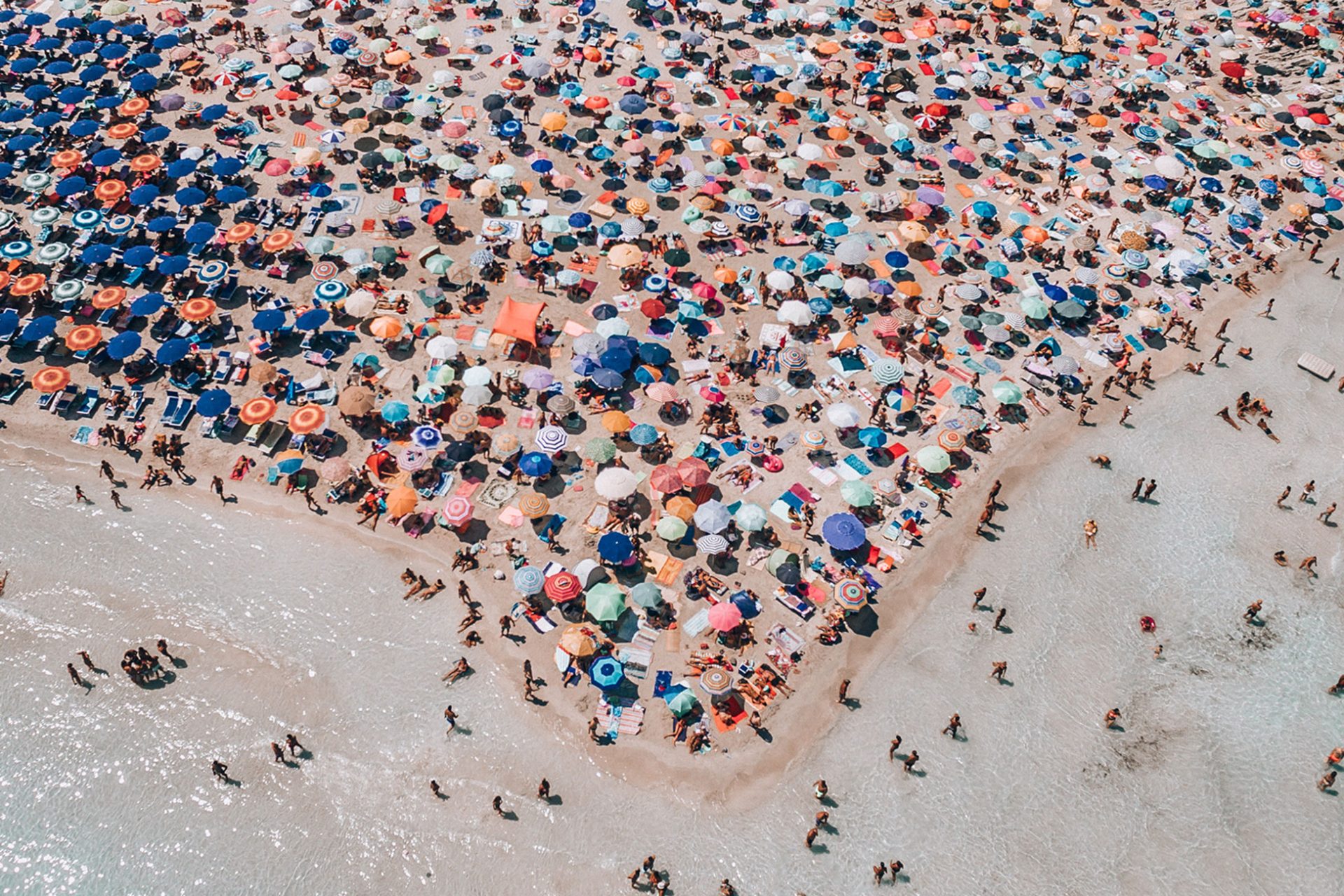An aerial photograph captures a bustling sandy beach on a sunny day. The scene is dominated by an overwhelming number of beach umbrellas and people, making the beach appear almost entirely covered. On the left side of the image, numerous dark blue umbrellas are organized into neat rows. In contrast, as you look towards the right, the umbrellas become more scattered and diverse in color, featuring light pastel blues, pinks, whites, purples, reds, and oranges, including some striped patterns.

The shoreline curves gracefully from the upper left, down towards the center, and back up towards the upper right of the photo. The ocean water is crystal clear, with many beachgoers wading, swimming, and walking along the beach. The sandy beach has a clean appearance, though it is densely populated with people, umbrellas, and various beach towels spread out across the sand. The detailed view from this high altitude makes the individuals look as small as ants, highlighting the vast occupancy of this very crowded beach.